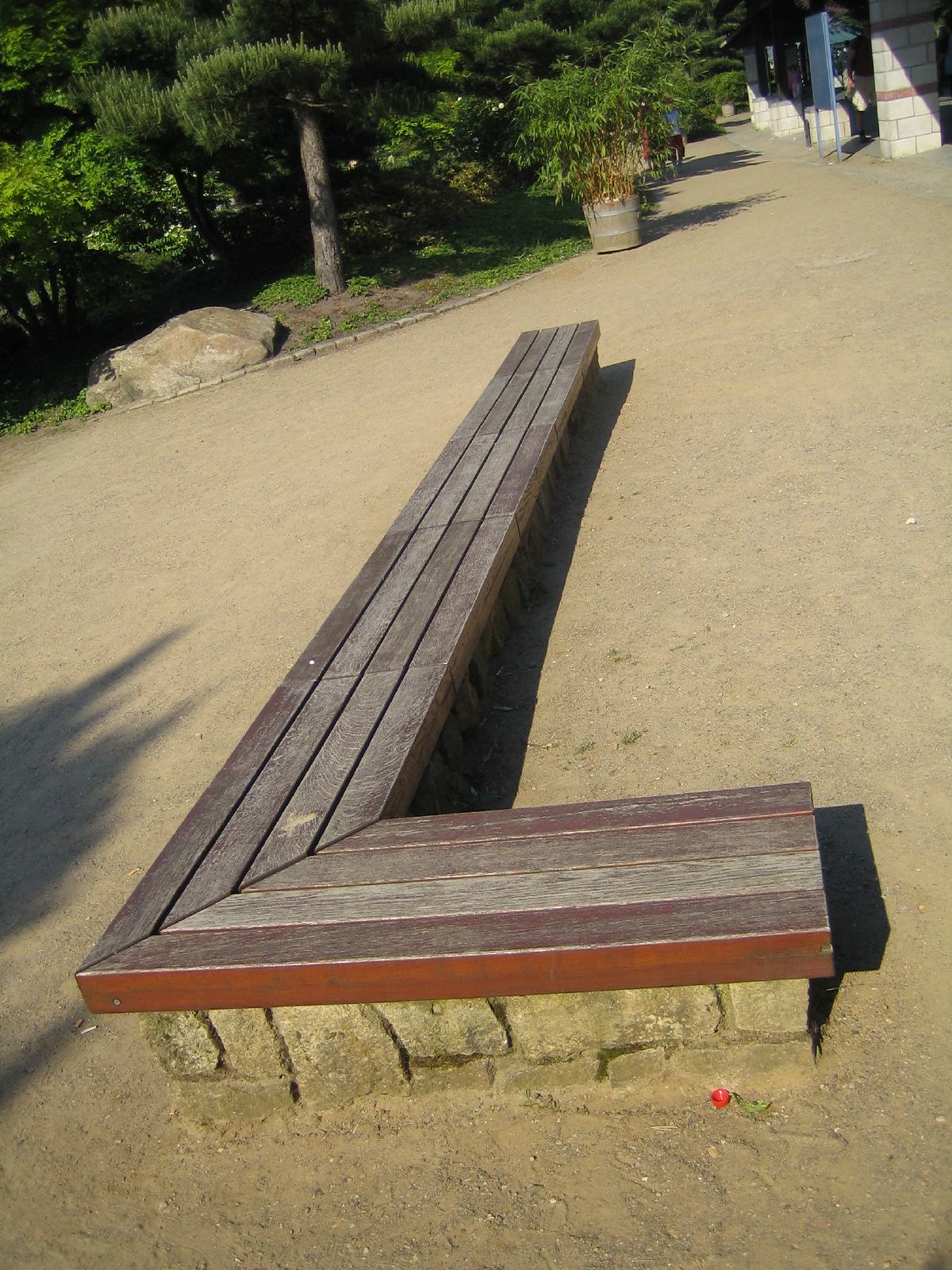The image captures an outdoor garden scene during the day, characterized by a mix of natural and constructed elements. The focal point of the image is an L-shaped bench with a seat made from brown-painted wood, sitting atop a stone base. The bench has a distinctive 90-degree angle and is set on a flat dirt field, which is light brown in color.

To the upper left, there is a forest-like area filled with bright green trees and various bushes. In front of this area lies a very large stone on the grass. Along a dirt and gravel walkway, which is separated from the grass by bricks, you can see multiple wooden containers with potted plants. There is also a conspicuous large flat rock and what appears to be a little red object resembling a half eggshell sitting next to a pile of stones.

In the upper right corner, there are several people near a building with white bricks. One person is wearing a black shirt and white shorts, while others are clad in pink and light blue dresses. The building features brick pillars and a big blue sign, possibly a directory, and there appears to be an entryway where tickets might be purchased. The overall scene is lush with greenery, including sharp-pointed leaves and various forms of shrubbery, giving the place a vibrant garden-like atmosphere.